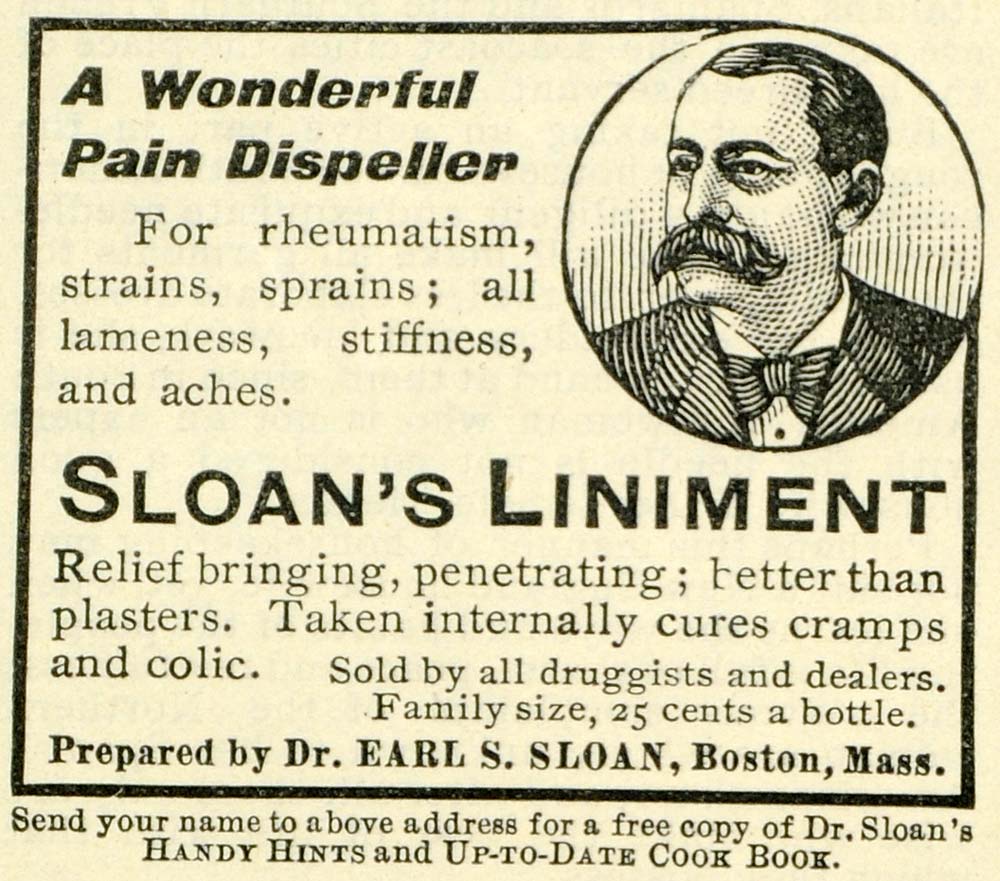This image is an old advertisement, likely cut from a yellowed newspaper. The background features a light tan color indicative of aged paper, and all the text is in bold black print, primarily in capital letters for emphasis. Dominating the ad is the headline "A WONDERFUL PAIN DISPELLER," followed by the claims: "for rheumatism, strains, sprains, all lameness, stiffness, and aches." The centerpiece is the product name, "SLOAN'S LINIMENT," under which it boasts to be "relief bringing, penetrating, better than plasters." Additional information states that it can be "taken internally, cures cramps and colic." The product is described as sold by all druggists and dealers, available in a family size for 25 cents a bottle, and is prepared by Dr. Earl S. Sloan from Boston, Massachusetts. In small print, the ad invites customers to send their name to the provided address for a free copy of "Dr. Sloan's handy hints and up-to-date cookbook."

In the upper right corner of the ad, encased within a circular border, is a black-and-white line drawing of a man with a large bushy mustache, dark hair, and a suit with a bow tie, likely Dr. Earl S. Sloan himself. The detailed illustration and formal attire suggest a man of prestige and trustworthiness, enhancing the advertisement's credibility.